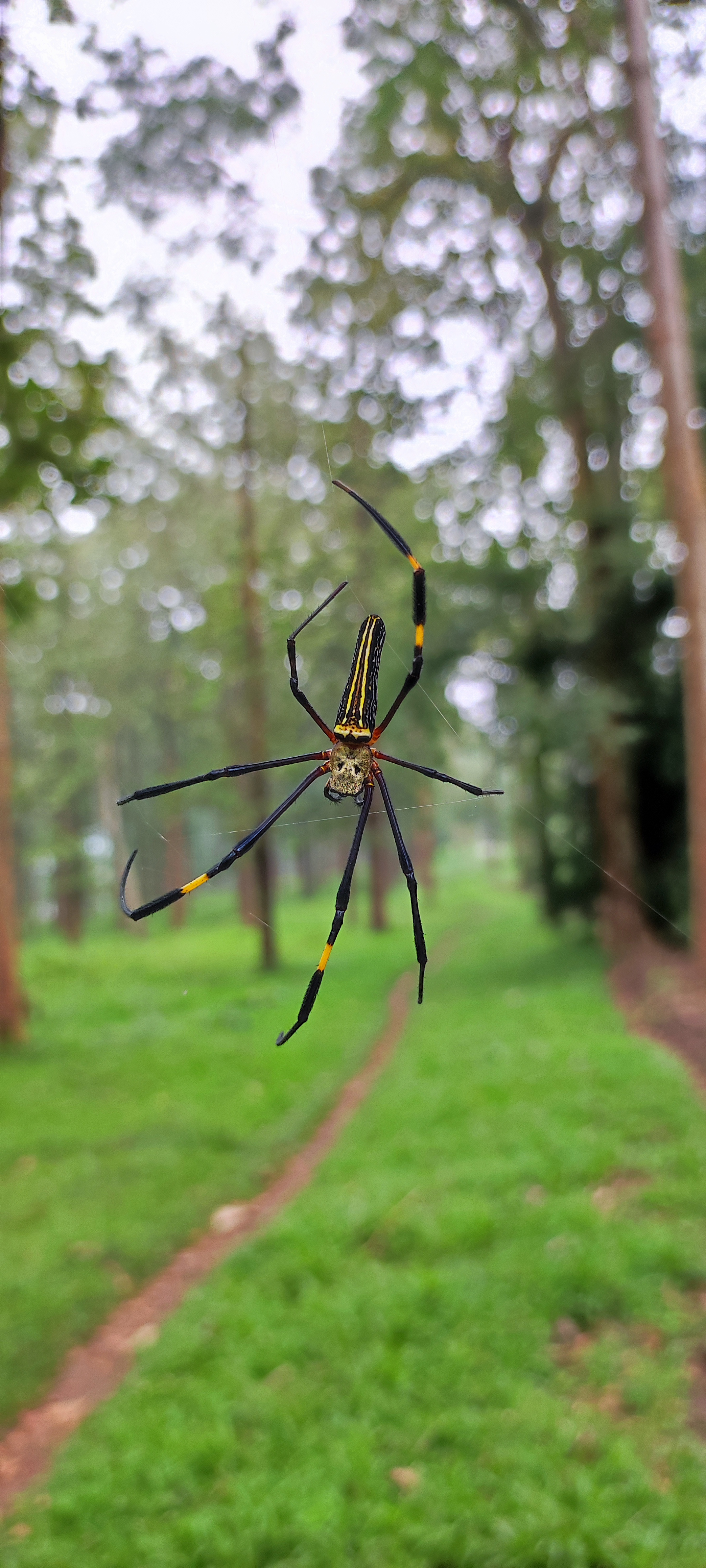This close-up image captures a Japanese orb-weaver spider, now considered an invasive species in America. The spider’s elongated, cone-shaped abdomen is predominantly black, marked with two distinct yellow stripes. Its legs are long and slender, primarily black with several yellow rings encircling them. The head is a large grayish-white, almost skeletal in appearance, with visible mandibles. The spider is suspended on its web, which is nearly invisible, giving the impression that it’s floating midair. The background features a brightly lit forest trail with trees and grass flanking a narrow dirt path, but the spider remains the main focus of the image, standing out starkly against the blurred foliage.